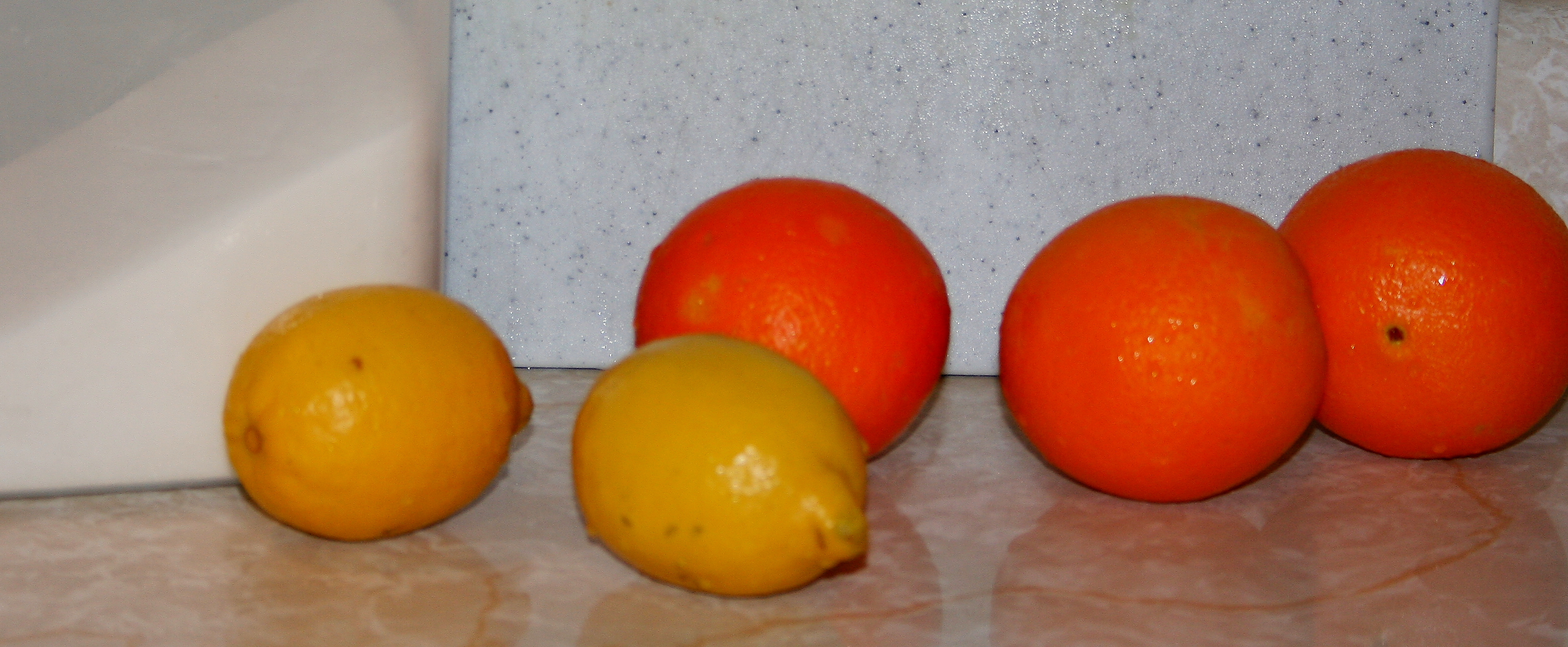The image features five pieces of fruit arranged randomly on what appears to be a marble countertop. Three of the fruits are pristine, vibrant oranges, while the remaining two resemble slightly bruised lemons with yellowish skin. The background showcases a contrasting surface, possibly a different style of tile or the edge of the countertop, highlighting the fruits vividly against the varied textures. The clean, unblemished appearance of the oranges stands in stark contrast to the mildly marked lemons, creating a visually appealing and detailed composition.